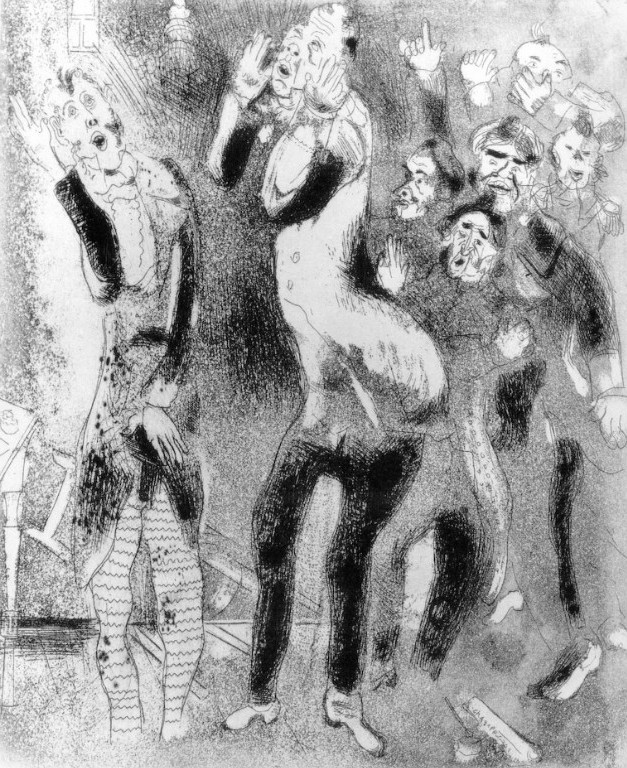The black-and-white drawing, possibly created with pencil or charcoal on paper, presents a highly stylized and abstract scene of several people, predominantly men, with elongated, wavy bodies and distorted faces. The foreground features two men, seemingly the primary focus, who might be performing or singing. The man on the left is notable for his black jacket, white shirt, and zigzag striped pants, while the man on the right wears a white jacket, black pants, and white boots. Their darkly shaded arms emphasize their old-fashioned long coats. Surrounding them is a chaotic crowd with fragmented, surreal body parts visible—such as just a leg, an arm, or fingers—creating a disjointed background. To the left, a partly visible writing table and a ladder are sketched, and on the bottom right, near some spectators, lies a piece of paper with writing and an inkwell filled with ink. Overall, the image exudes a surreal, unsettling atmosphere with its overlapping elements and abstract human forms.